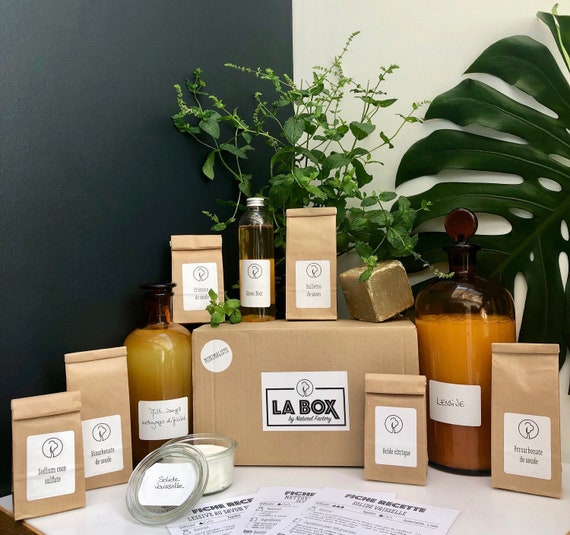The image showcases a detailed sales display for a series of L.A. Box products, prominently featuring a central box with a white sticker reading "L.A. Box" in black bubble lettering, by an unknown entity with the initials "NF" and an indistinct logo, possibly a cloud or tree. The display includes various brown paper bags, each marked with the same logo and diverse product names. Surrounding the central box are two bags on either side and two atop it. The table holds numerous items including a large brown bottle of liquid, small containers potentially filled with hand and face creams, and transparent glass containers. In front of the box sits a yellowish-orange jar, alongside two similar jars flanking the box. Additionally, there are three pamphlets with black writing laid out on the white table.

The background enhances the aesthetic appeal, featuring a dark blue wall on the left and a white wall on the right. This is complemented by lush greenery, with a vine-like plant and a large tropical leaf providing a vibrant touch. The cohesive arrangement of the products, coupled with the thoughtfully curated decor, highlights the L.A. Box brand in an elegant and appealing manner.